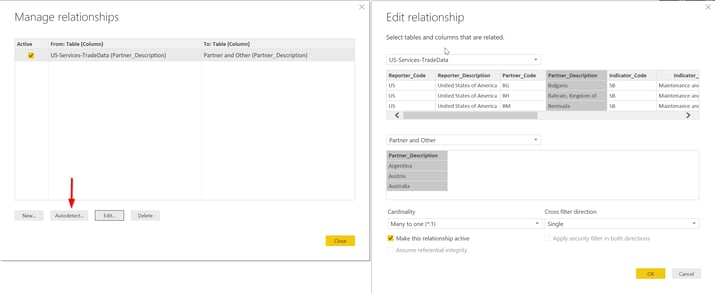**Image Caption:**

The image is divided into two sections. 

**Left Section:**
This section features a large gray-outlined square against a white background. Centered within the square, black-gray text reads "Manage Relationships." Below this heading, there are labels in black text on a gray background that say "Active," "From Table Column," and "To Table Column." A red arrow points downward within the square, leading to two buttons: a gray box labeled "Edit" and a yellow box labeled "Close."

**Right Section:**
The right side of the image also has a white background and features the heading "Edit Relationship" in gray text. Below this heading, a subtext in gray reads "Select Tables and Columns that are related." This section includes two tables filled with various entries in gray and black text. One of the tables has a scroll box, indicating that it can be scrolled horizontally. Additionally, there is a small yellow-highlighted square with a black check mark inside it. Towards the bottom, two buttons are visible: a small yellow rectangle with black text that reads "OK" and a gray rectangle with black text that reads "Cancel."